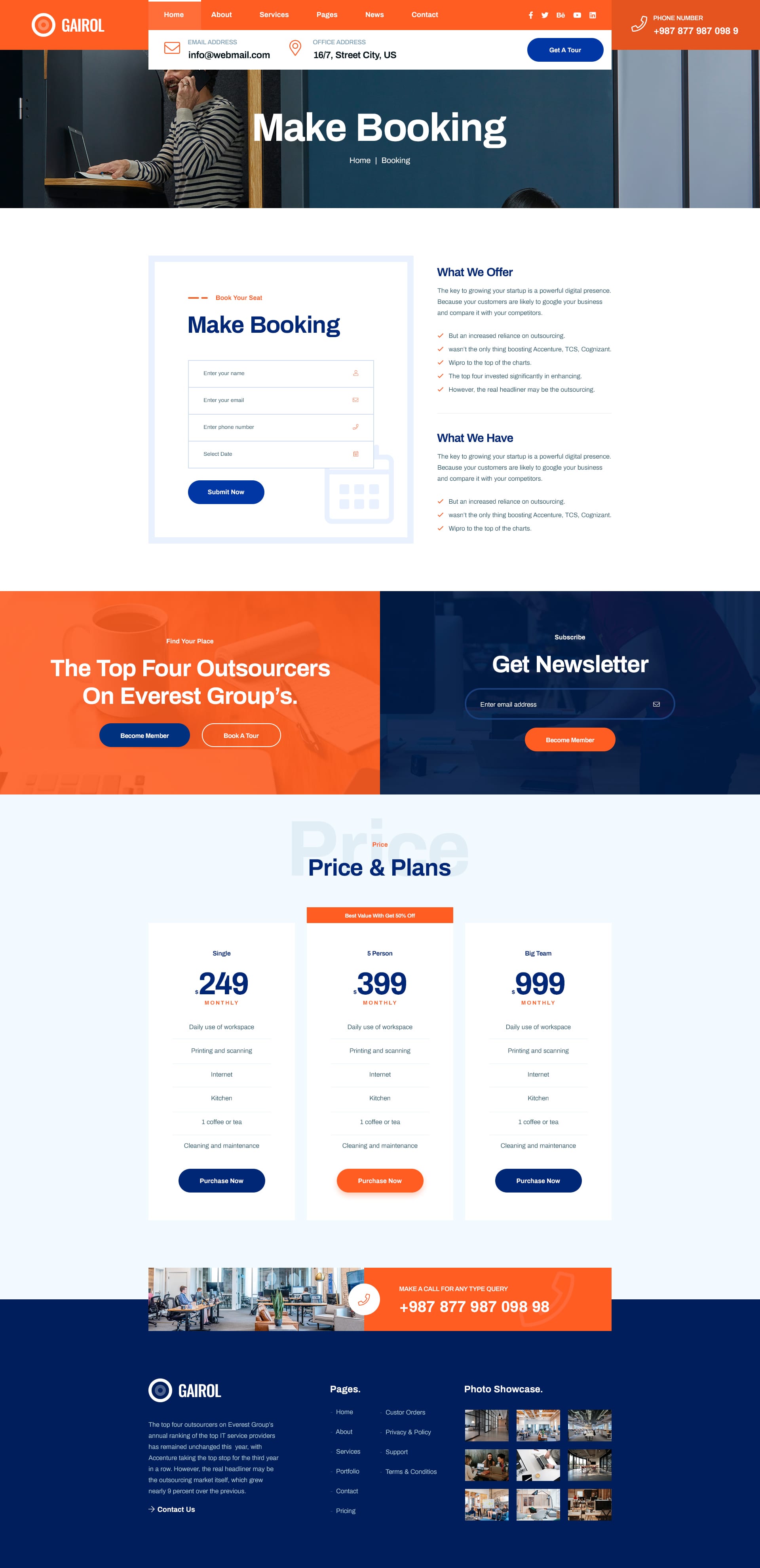This is a detailed description of the web page for booking:

At the top of the web page, there's a prominent orange banner. Directly below the banner, there's an image of a person standing at a computer desk using a laptop while holding a phone to their ear. Superimposed on this image, centered, is the text "Make Booking" in white letters.

Beneath the image, a series of boxes and squares are displayed, some featuring a white background with light blue outlines. The topmost box with a light blue outline contains the text "Make Booking" in blue lettering at the top.

Further down the page, around the middle, there is a distinctive banner split into two sections: the left side is orange, and the right side is dark blue. The orange section of the banner reads, "The Top Four Customers on Events on Everest Groups." In contrast, the right section of the banner displays the title "Get Newsletter" in white letters, alongside a blue entry form where users can input their email addresses.

Just below the middle of the page, on a white background, is a section with blue lettering that reads, "Prices and Plans." This section lists three different prices: the first price on the left is $2.49, the middle price is $3.99, and the price on the right is $9.99.